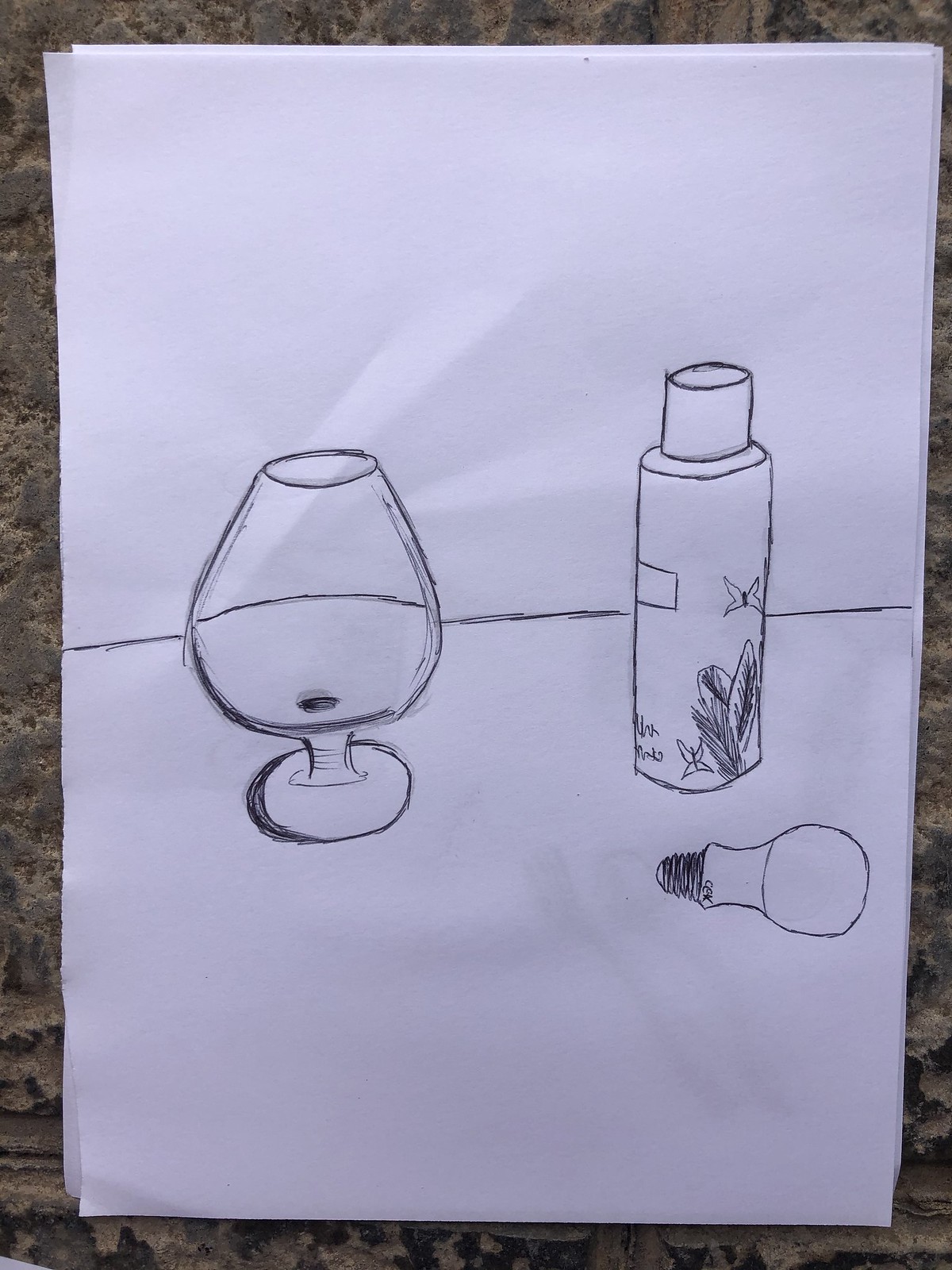This image showcases a meticulous hand-drawn artwork on a piece of white, wrinkled paper. On one side of the paper, a wine glass filled with liquid is prominently featured. Adjacent to this, a small light bulb is drawn, lying on its side with its metallic base clearly depicted. Next to the light bulb, there is an illustrated bottle adorned with a rectangular label on one side and a cap. The bottle artwork includes intricate details of a butterfly with a dark center, leafy embellishments below, and a smaller butterfly situated to one side of the leaves. Additionally, there is a section of black text beside the smaller butterfly, though the font is too diminutive to discern.